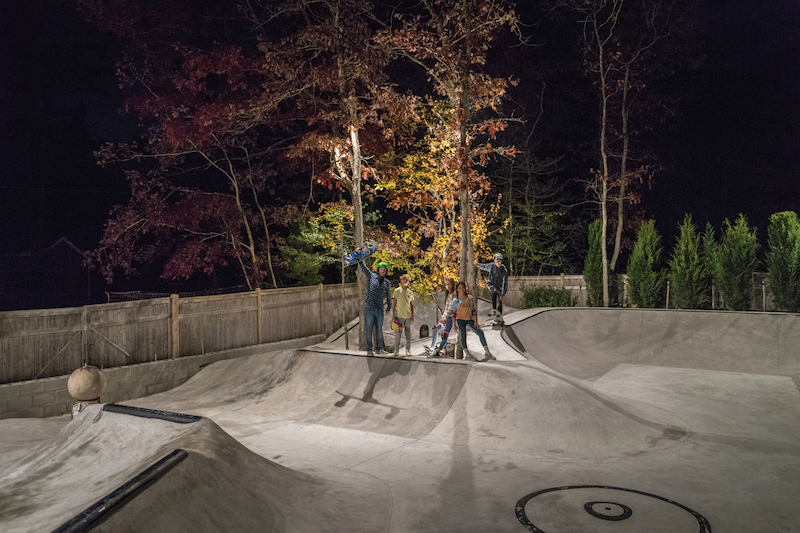In this detailed nighttime image of a skate park, five kids are seen at the top of various ramps, all wearing helmets and illuminated by a bright light from behind the trees. One child holds a skateboard triumphantly above his head, while another balances on his board. The remaining two girls grasp their skateboards in their hands, with a mix of red, orange, yellow, green, and purple leaves from fall foliage trees framing the scene. The smooth concrete park is dotted with grind bars and encircled by a wooden fence, creating a vivid composition against the dark black sky devoid of stars. Below the trees are shorter, evergreen shrubs, adding a touch of green to the autumnal landscape. The entire park, with its rock-like skateboard ramps and illuminated by a single streetlight, showcases a vibrant capture of youthful energy and the serene, colorful beauty of fall.